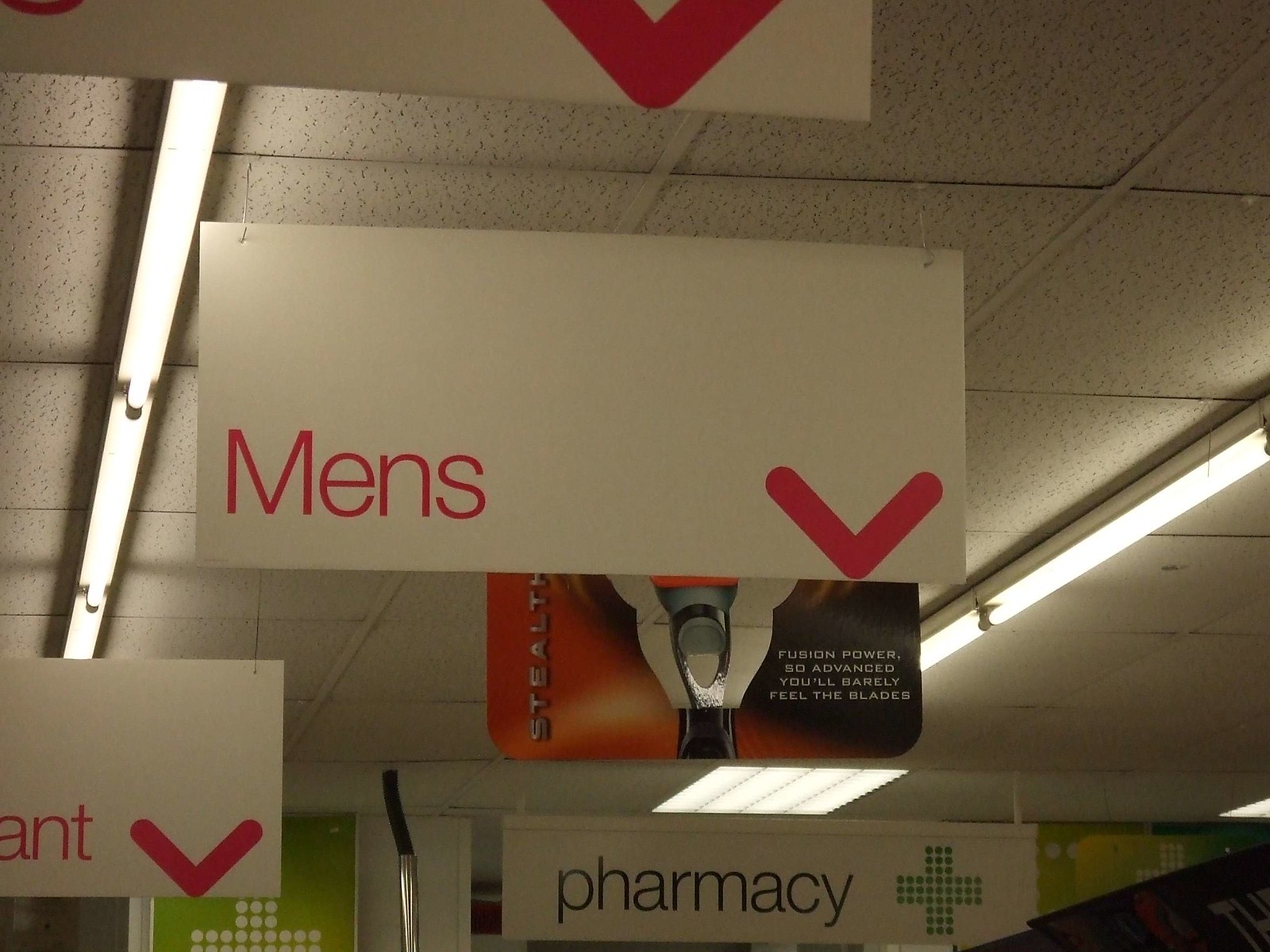The image depicts the ceiling of a retail store, likely a Target, characterized by its white tiled ceiling punctuated with small black spots and interlaced with white support bars and fluorescent lights. Several white signs with red text hang from the ceiling. One prominent sign reads “Men's” with a downward arrow pointing to the men's section below. Another sign, partially visible, seems to read “Infant”, represented only by the letters “Ant” and a similar downward arrow. In the foreground, a large white sign advertises the “Fusion Power 3D Advanced” razor blade, promising an advanced, nearly imperceptible shaving experience, with the word “Stealth” on the left side in silver lettering. This sign also features a large image of the shaver. In the background, a distinct white sign with black text reads “Pharmacy”, accompanied by a green cross to the right, indicating the pharmacy section. This intricate display of signs, combined with the distinctive lighting and layout, suggests a well-organized store section likely dedicated to personal care and hygiene products for different demographics including men, women, and infants.